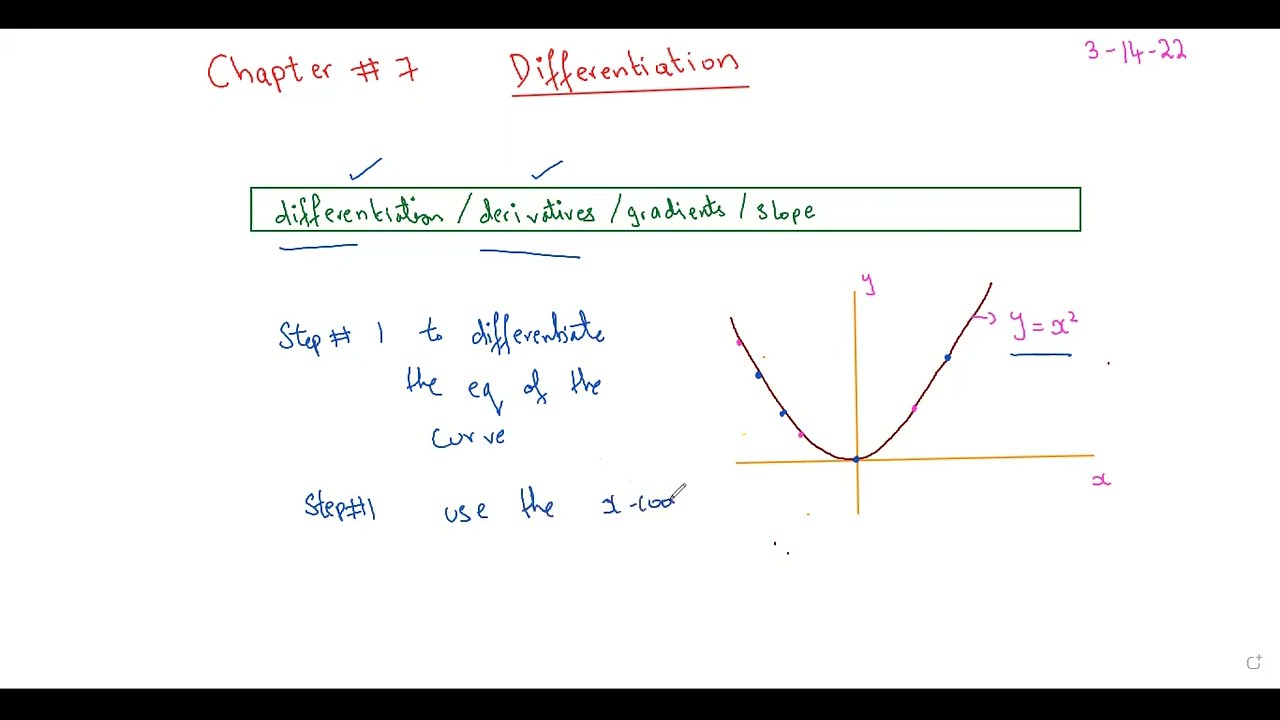This image features a whiteboard with a detailed mathematical presentation. At the top left in red letters, it reads "Chapter 7: Differentiation," with "Differentiation" underlined. In the top right corner, the date "3-16-22" is noted. Below the title, there is a small green rectangle containing the terms "Differentiation / Derivatives / Gradients / Slope," with "Differentiation" and "Derivatives" each marked by a blue checkmark. Further down, in blue writing, it states: "Step number 1: To differentiate the EQ of the curve. Step 1: Use the SL/cool." Off to the right side of the board, there is a graph depicting a U-shaped curve (a parabola) with the equation "Y = X²,"  highlighted in pink and underlined in blue.